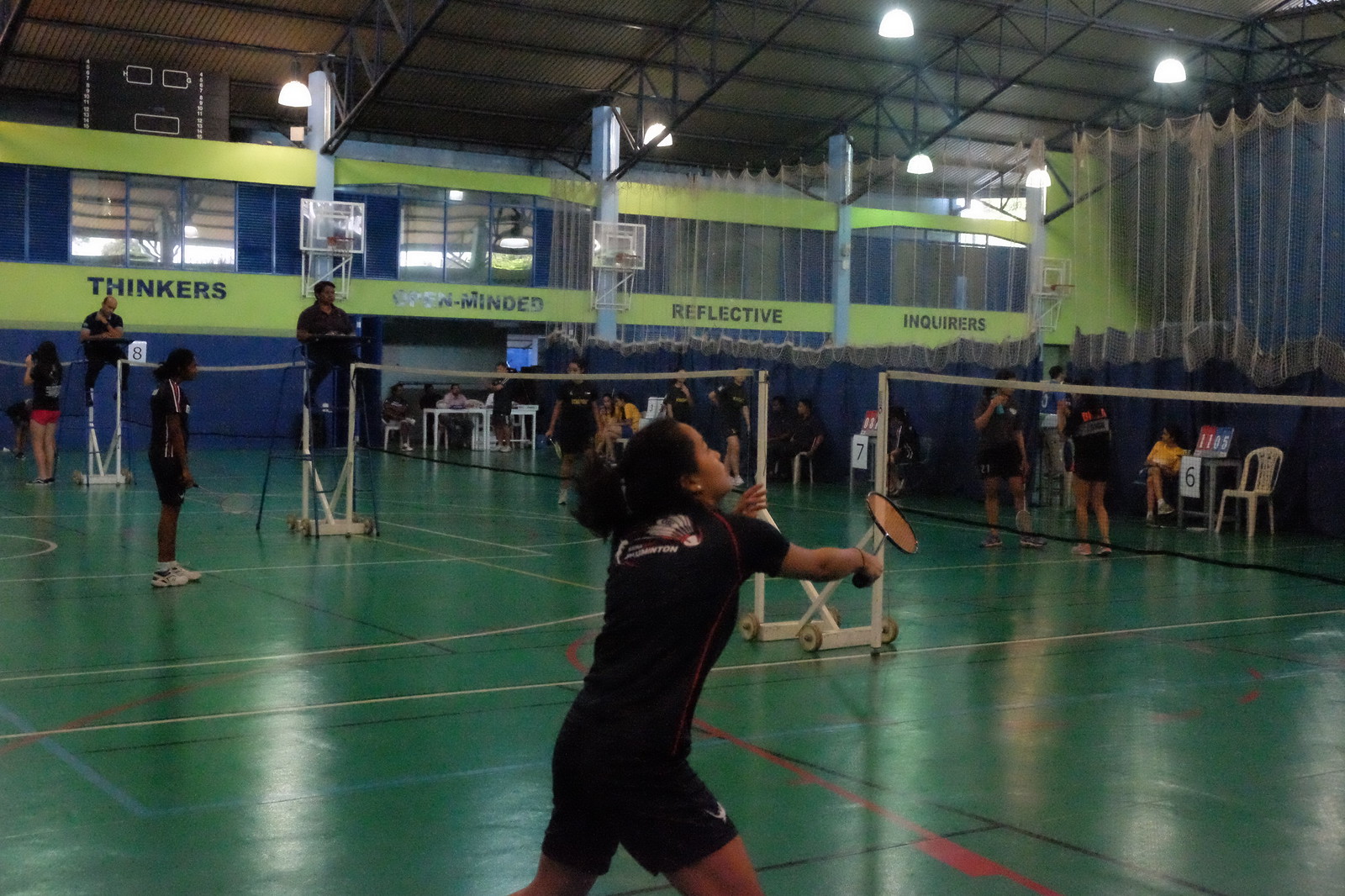The photograph captures an indoor sports event, specifically a badminton match set up within a multi-purpose gym. Dominating the foreground is a woman dressed in a black uniform, her dark hair tied back in a ponytail. She is captured in a dynamic pose, either having just hit or about to hit a badminton shuttlecock, her racket extended in her hand. Viewed from the side, the focus is on her shoulder, and only a partial profile of her face is visible. The green floor is marked with various colored lines—black, white, red, and blue—indicating different sports boundaries.

Multiple badminton nets are set up across the court, with referees positioned on high chairs at the ends of the nets, overseeing the matches. In the background, the right wall showcases a second story with large windows, allowing natural light to filter into the gym. A sign on the wall reads "Thinkers, Reflective, Inquiries." Along this wall, a mix of seated and standing spectators are visible, observing the ongoing matches. The ceiling’s framework and hanging lights complete the scene, highlighting the indoor setting of this versatile sports facility.